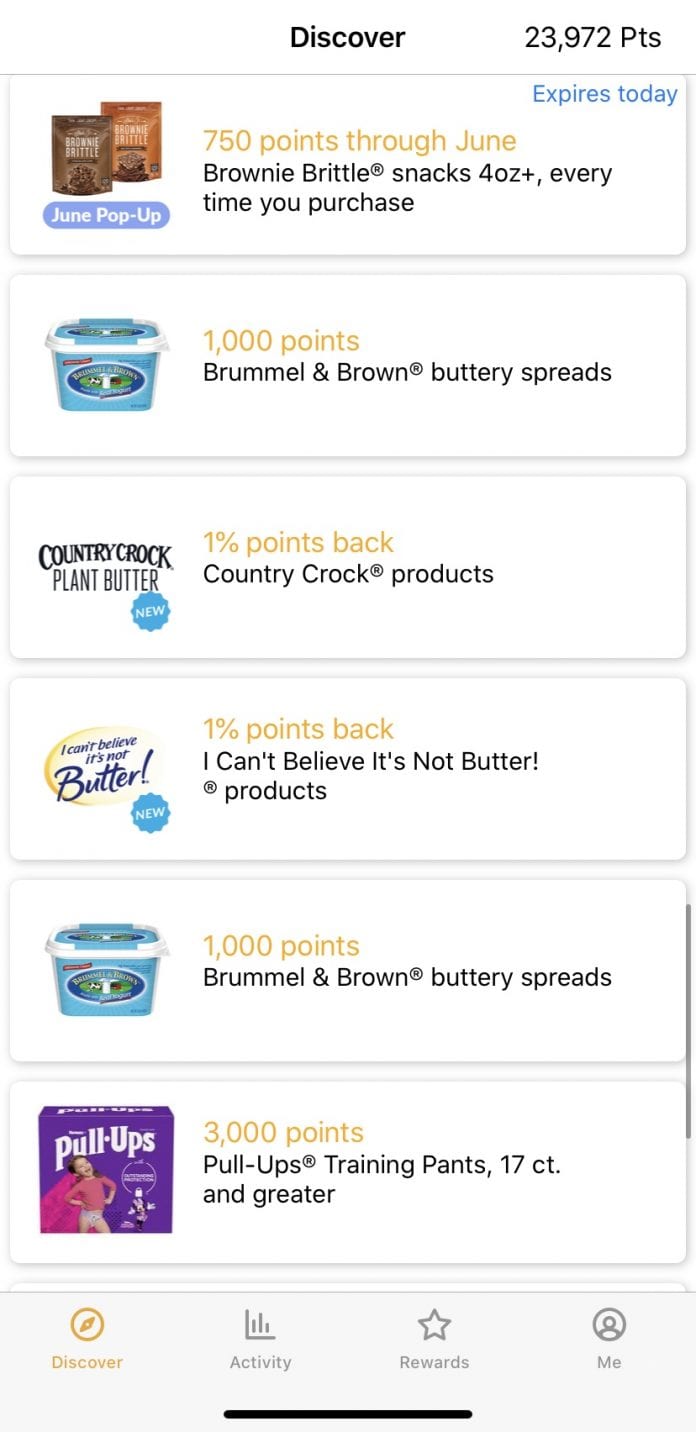The image showcases an assortment of grocery products under a banner that reads "Discover," alongside an impressive tally of 23,972 points. The background is predominantly white, framed by rows of gray boxes that neatly categorize each item.

- The first row features two varieties of Brownie Brittle. The left bag is dark brown, and the right is light brown, each displaying an appetizing image of the brownie brittle inside.
- Moving down, the next product is Brummel and Brown Buttery Spreads, packaged in a blue tub with white trim. A circular graphic at the center depicts a cow, possibly accompanied by a silo and barn.
- Following that is Country Crock Plant Butter, distinguished by a star-shaped emblem labeled "NEW." The package has a blue design with white lettering.
- Next in line is "I Can't Believe It's Not Butter" with its iconic blue script set against a yellowish, round backdrop fashioned in a swirling pattern.
- Another Brummel and Brown Buttery Spread appears next, identical to the first with its blue tub and white trim, again featuring the prominent cow graphic.
- The final product is Pull-Ups Training Pants, housed in a vibrant purple box. The box showcases a toddler in a pink short-sleeved T-shirt and the training pants, who also sports a pink superhero cape, adding a playful touch to the packaging.

This descriptive arrangement provides a detailed overview of the diverse grocery selections presented in the image.